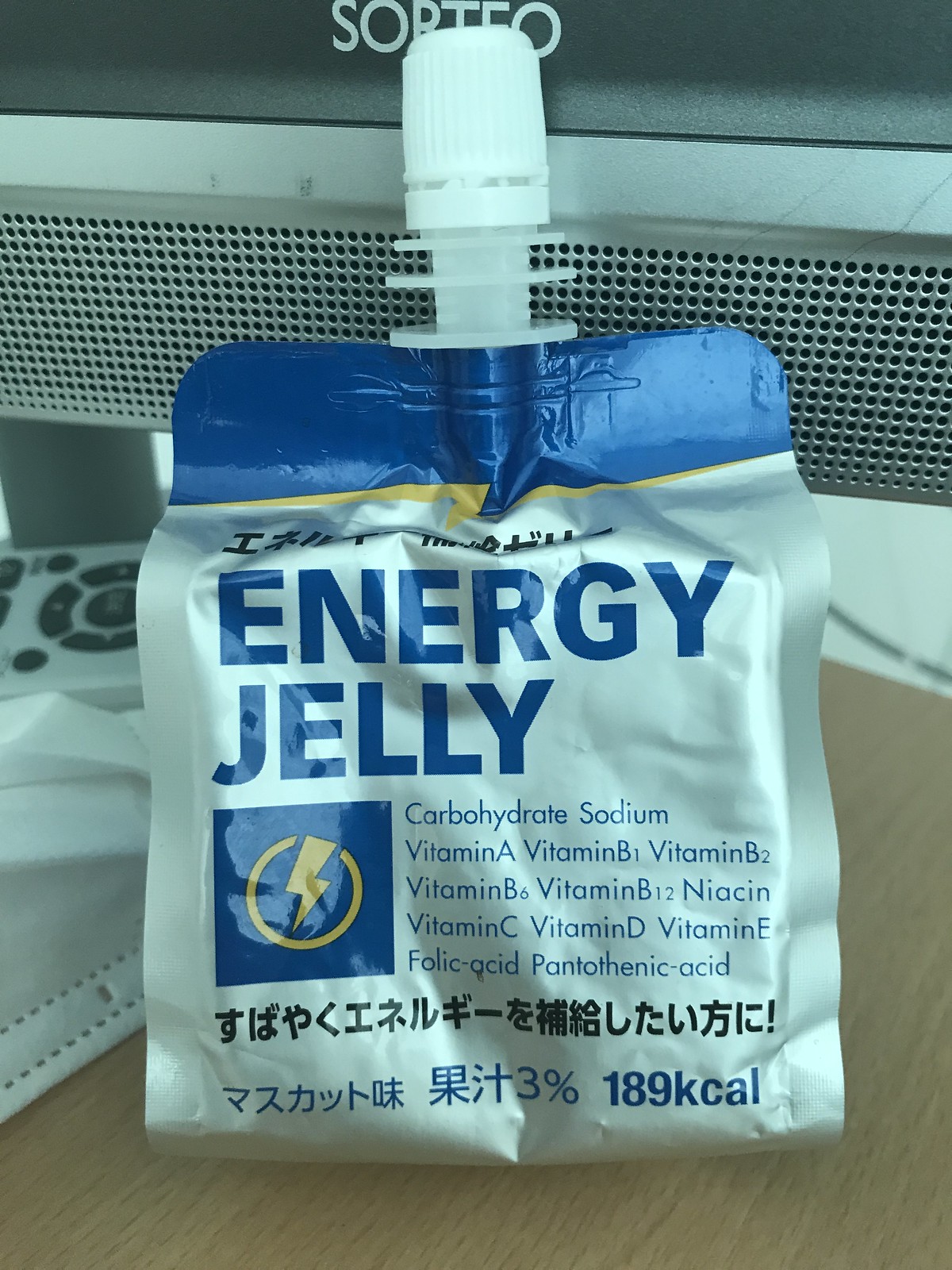This photo features a square-shaped product package with a sleek, silver exterior. The packaging prominently displays "Energy Jelly" in bold blue lettering. A striking blue square with a yellow lightning bolt emerges from the center, symbolizing energy and vitality. At the top, a solid blue band adds contrast and visual appeal. Detailed nutritional information is provided, highlighting ingredients such as hydrate, sodium, vitamin A, and various B vitamins. The bottom of the package notes a caloric content of 187 kcal. Surrounding the main text are numerous characters in an Asian script, suggesting that this product is likely marketed in an Asian country. The package rests on a brown table, with a remote control positioned behind it, possibly indicating a TV setting.